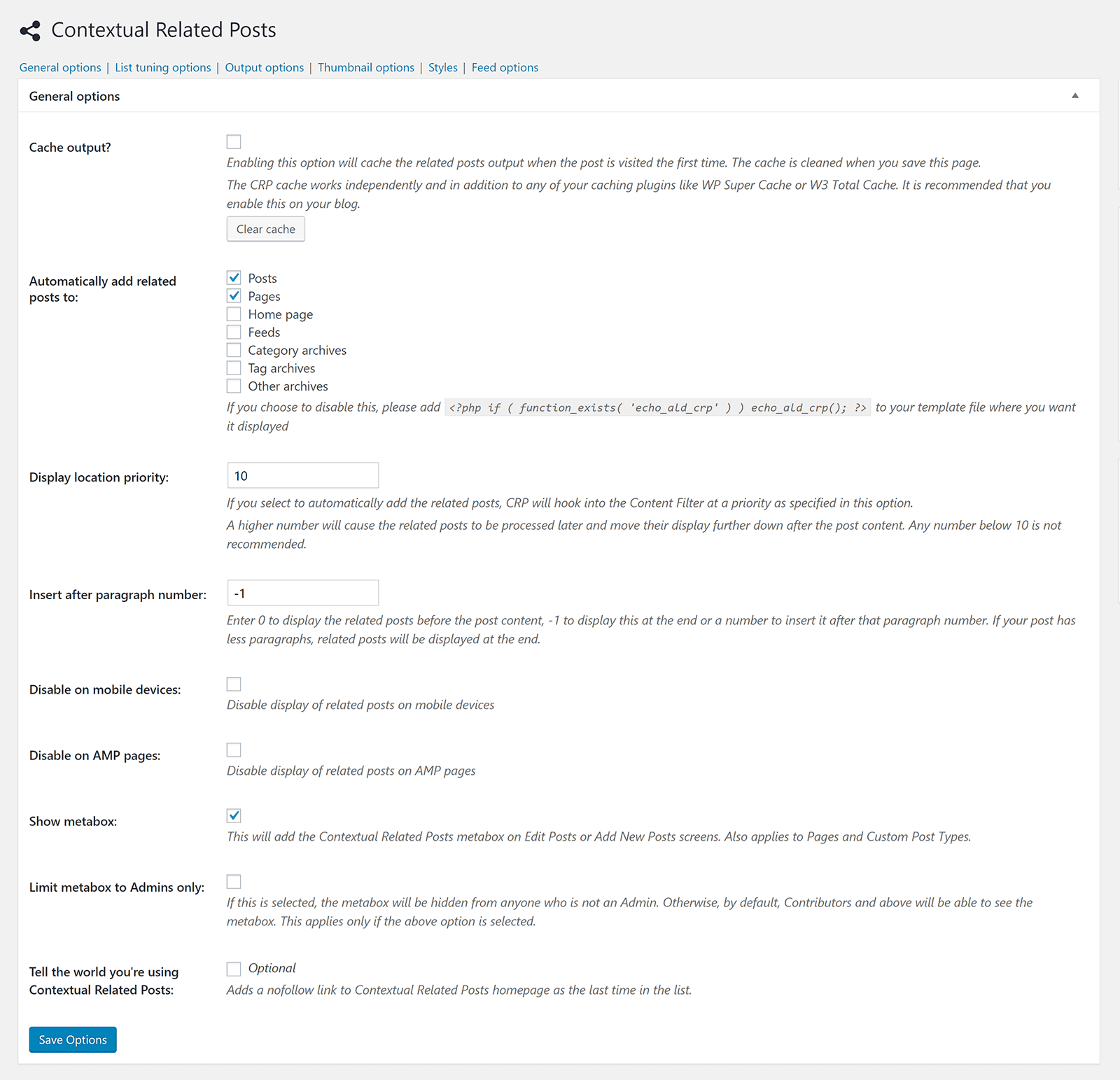Here's a detailed and cleaned-up caption for the described image:

---

The image appears to be a screenshot of a settings page from a website or application, most likely related to a Content Management System (CMS) like WordPress. The page is framed by a light grey border, and a top light grey bar contains the section title "Contextual Related Posts" written in black text.

Below this title, various sections are listed in a vertical layout, including:

- **General Options**
- **List**
- **Tuning Options**
- **Output Options**
- **Thumbnail Options**
- **Styles**
- **Feed Options**

Inside the "General Options" section, several settings are described in detail:

- **Cache Output:** A checkbox that can be toggled on or off. The accompanying italicized explanatory text advises, "Enabling this option will cache the related posts output when the post is visited for the first time. The cache is cleared unless you save the page. The CRP cache works independently of any other caching plugins like WP Super Cache or W3 Total Cache. It is recommended to enable this on your blog."
- **Automatically Add Related Posts to Posts and Pages:** This is followed by checkboxes for various categories:
  - **Home Page:** Unchecked
  - **Feeds:** Unchecked
  - **Category Archives:** Unchecked
  - **Tag Archives:** Unchecked
  - **Other Archives:** Unchecked
  
  A note suggests that if automatic addition is disabled, users must manually insert a block of provided computer code into their template where they want the related posts to display.

- **Display Location Priority:** Currently set to 10, with further instructions below this setting.
- **Insert After Page Number -1:** Includes additional instructions for proper usage.
- **Disable on Mobile Devices:** Unchecked, with supplementary instructions beneath.
- **Disable on AMP Pages:** Unchecked, with additional guidance provided below.

Further settings include:

- **Show Meta Box:** Checked. The description explains that this will add a meta box for contextual related posts in the edit passage or add new post screens, also applicable to pages and custom post types.
- **Limit Meta Box to Admins Only:** Unchecked, with more instructions beneath.
- **Tell the World You're Using Contextual Related Posts:** Optional and unchecked, followed by instructions.

At the bottom left corner, there’s a blue "Save Options" button with white text, although the text throughout the page appears somewhat distorted and poorly rendered.

The screenshot demonstrates a comprehensive configuration interface with extensive options for tailoring how related posts are managed and displayed on a website.

---

This detailed caption should provide a clear and thorough description of the screenshot, reflecting both its layout and content.